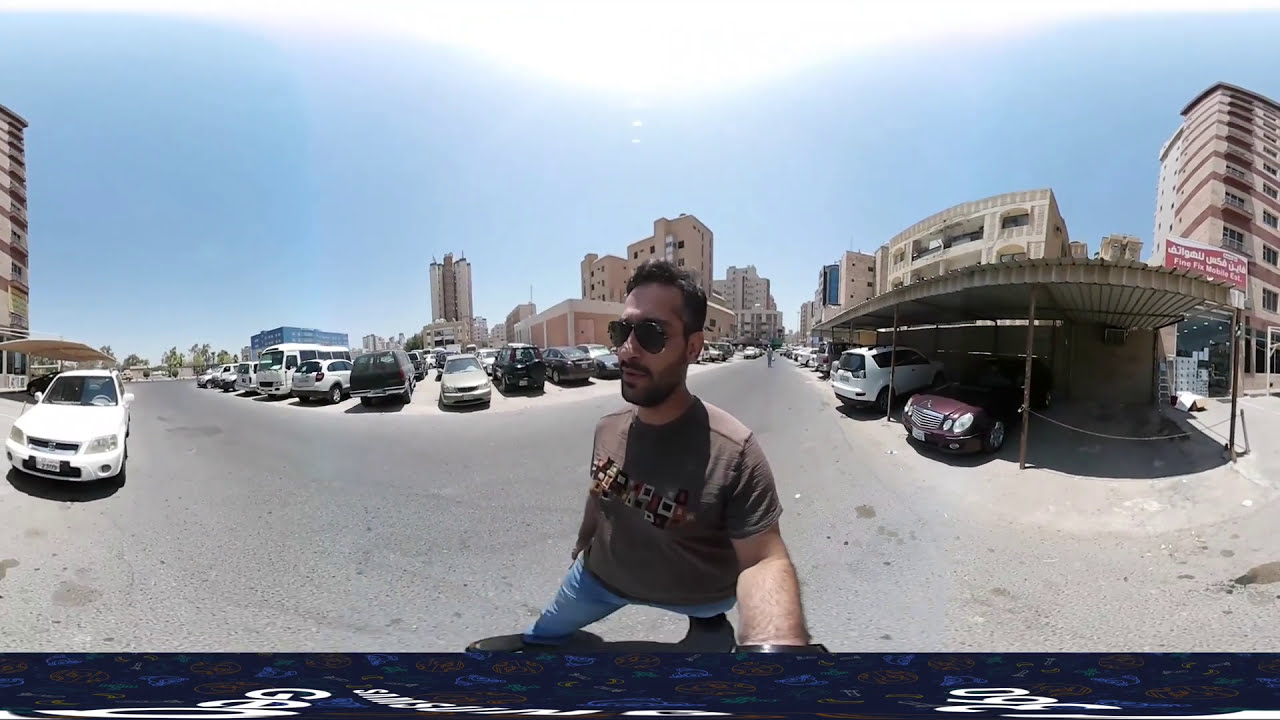A man with black hair and dark sunglasses stands on a city street, appearing to use a selfie stick to take a picture of himself. He is dressed in a brown short-sleeve shirt, light blue pants, and has a leather-colored strap around his wrist. The street beneath him is light gray, and he is staring towards the left. Directly behind him is a tall, brown building with square windows, and just to its left is another tall building with a darker brown center. To the right, there is a carport sheltering a white van and a maroon-colored small car; one parking space is blocked off by a hanging rope. Additionally, a nearby multi-story building transitions from dark brown to light brown and has windows on every floor.

The background is bustling with numerous cars, including a red one, several white ones, a silver one, a gold one, a black one, and even a bus. Many cars are parked in a sunlit dirt parking lot, though a few are under an awning to shield them from the intense sun. The sky is blue, with a bright white light in the center, showing a slight green tint around its edges. The scene appears to be set in a non-American, possibly European, urban area that feels laid-back and relaxed. The man seems to be sweating, hinting at warm weather. There's also an oil stain in the bottom right corner of the image, indicating a well-used thoroughfare.